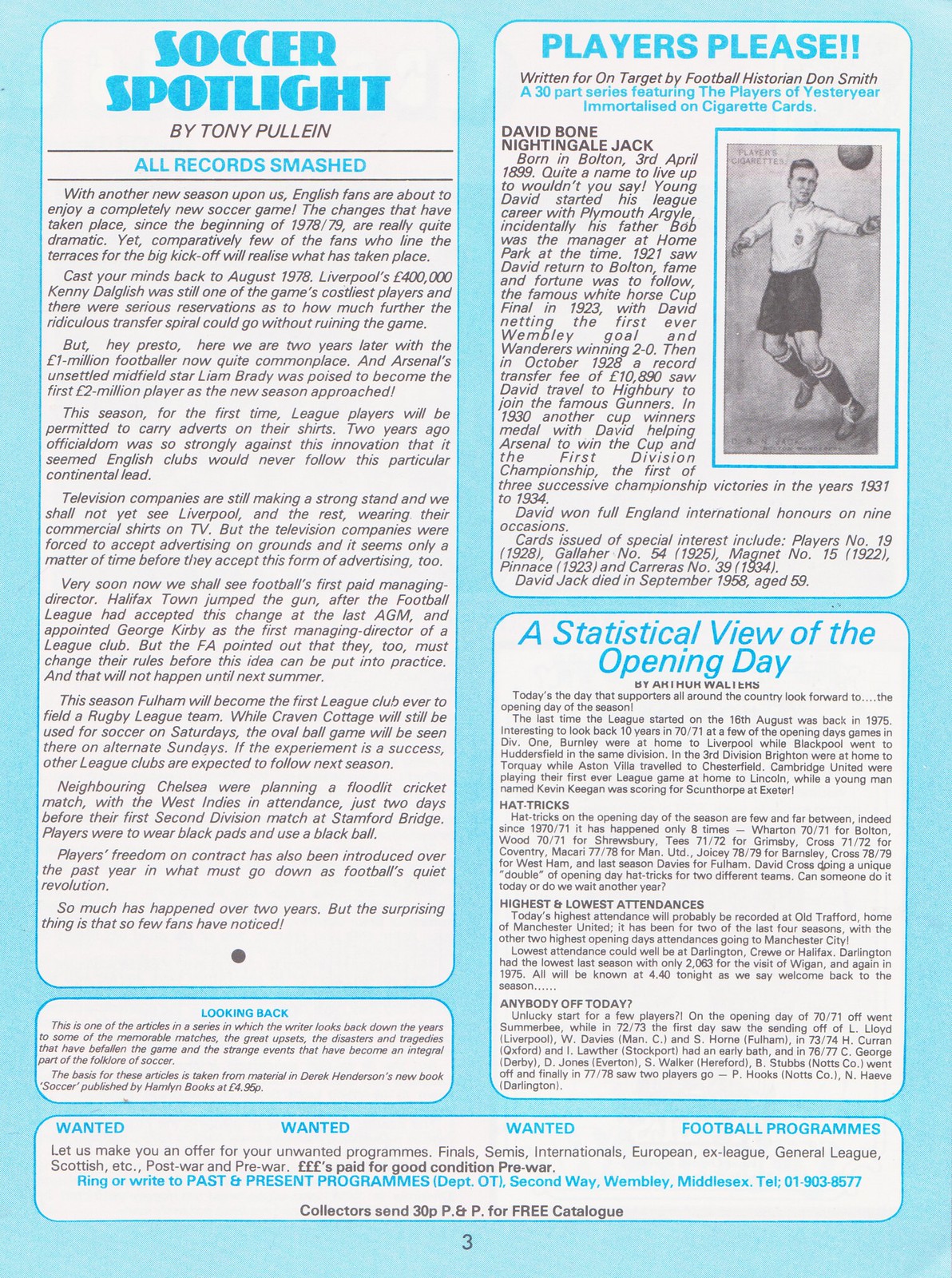This image captures a detailed overview of a vintage magazine page titled "Soccer Spotlight" by Tony Pullian. The page, with a distinctive blue background and page number three at the bottom, features three major articles housed in white box sections with blue headings and black text. The main highlighted article, "Soccer Spotlight," discusses the dramatic changes in English soccer since the 1978-79 season, noting the hefty player transfers, including Liverpool's £400,000 Kenny Dalglish and Arsenal's Liam Brady nearing a £2 million move. It also touches on the new trend of league players carrying advertisements on their shirts and other significant shifts within the sport. Below this, in a smaller white box with the heading "Looking Back," the article reflects on memorable soccer matches and events, sourcing from Derek Henderson's book “Soccer.” Adjacent to this, a wanted ad for football programs sits prominently, emphasizing "Wanted, Wanted, Wanted Football Programmers" in blue text. On the top right portion, another article titled "Players, Please," by football historian Don Smith, details the career of David Owen Nightingale Jack, immortalized on cigarette cards. Lastly, the bottom right article provides "A Statistical View of the Opening Day" by Arthur Walters, offering insights and historical comparisons of league season openers, focusing on attendance figures and notable player performances. Overall, this magazine page is a comprehensive and nostalgic look at the evolving landscape of soccer during that era.